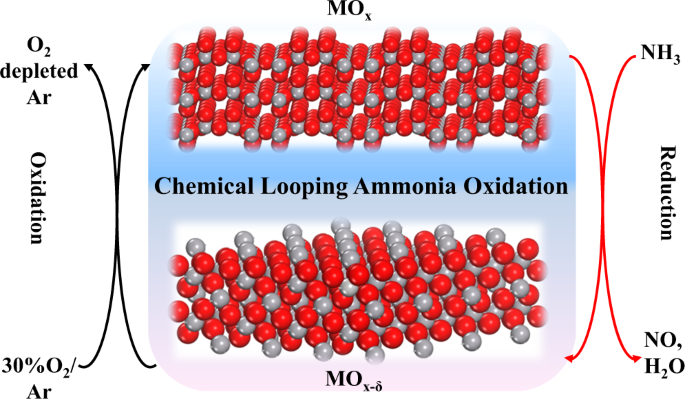The image is a detailed diagram on a white background, depicting the chemical looping process of ammonia oxidation. Central to the diagram, the phrases "chemical looping," "ammonia oxidation," and "MOX" are prominently displayed, with MOX possibly denoting a specific chemical formula or compound. The diagram features interconnected red and gray circles or beads, arranged in rows and patterns that resemble chemical bonds or capsules, often directed in a diagonal fashion.

On the left side, labels indicate "O2 depleted air" and "oxidation 30% O2 air," with black arrows directing attention to these stages. The central part of the diagram highlights the gray and red tubular structures, apparently undergoing oxidation and reduction reactions, further annotated with labels like "NH3" (ammonia) and "reduction NO, H2O." These labels are reinforced with color-coded arrows, including light blue, hazy purple, and red, pointing towards various stages and elements of the process.

Throughout the diagram, scientific equations and terms are scattered, explaining the intricate processes involving O2, NH3, and other compounds like NO and H2O. The interconnected beads, arrows, and labels collectively illustrate the elaborate chemical pathways and transformations involved in the ammonia oxidation reaction.